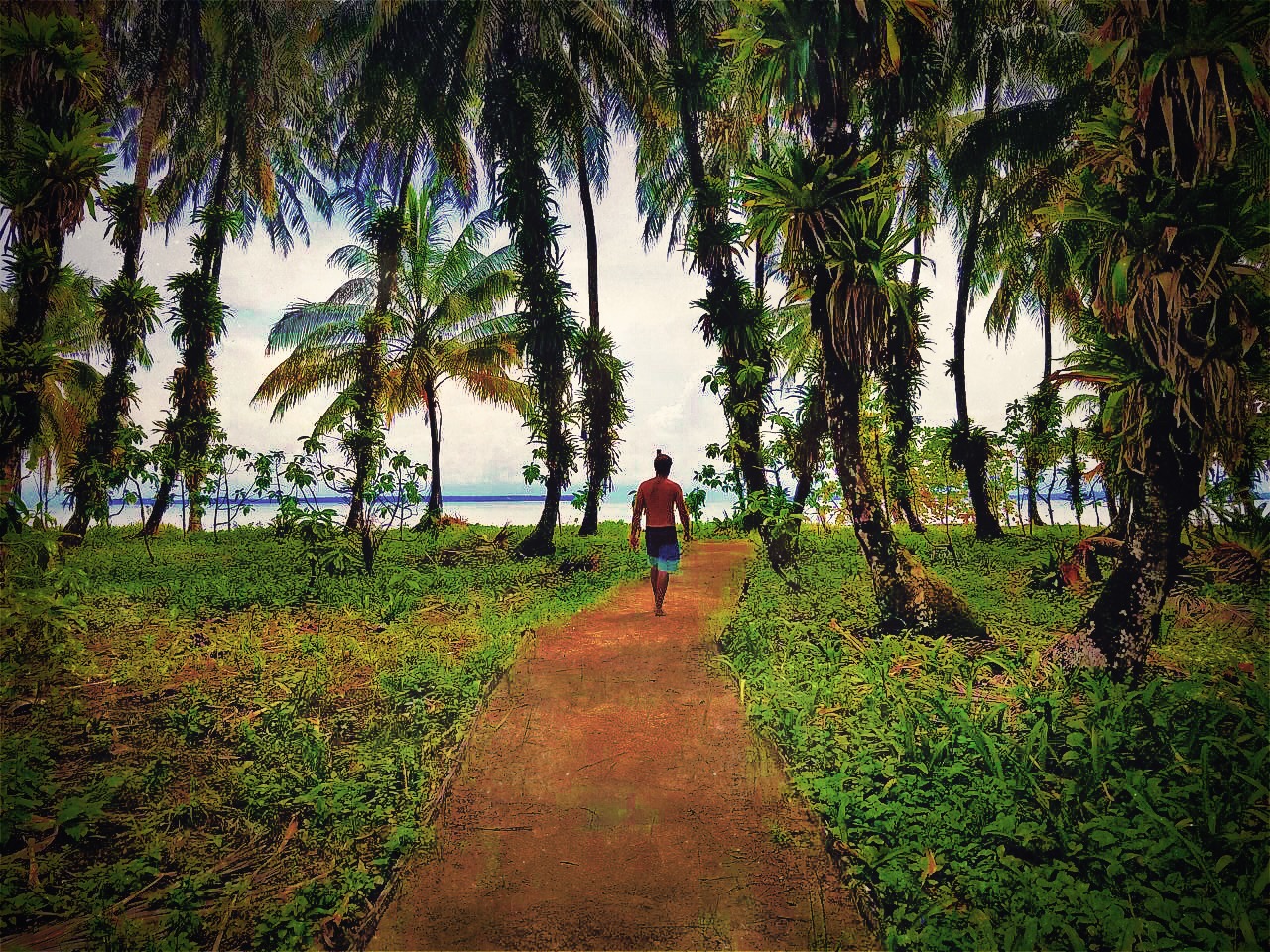The image captures a serene tropical pathway leading to a stunning beach scene. The central path, composed of reddish-brown soil and lined with leaves, cuts through lush greenery and vegetation. Tall palm trees flanking the path provide a dappled shade, creating a speckled light effect on the ground. About halfway down the path, a man with dark complexion, possibly of Asian descent, is visible from behind. He is shirtless, sports blue shorts that gradient from almost black at the top to teal at the bottom, and has his black hair styled in a bun. As he walks barefoot towards the beach, the distance reveals a white sandy shore meeting a blue, increasingly darker horizon. Overhead, the sky is overcast with light grayish-white clouds, adding a calm, tranquil mood to the midday or early morning scene. The photo exudes the peaceful allure of a tropical getaway, capturing both the dense foliage and the inviting ocean beyond.